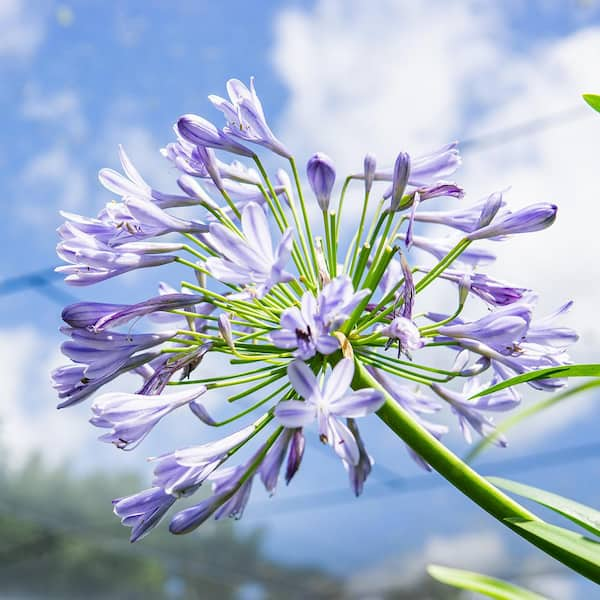This is a professional, square-shaped wildlife photograph featuring a stunning close-up of a flower, likely belonging to the Allium family. The central flower boasts a big, spherical flower head made up of numerous individual purple florets in various stages of bloom—some still in bud, others partially open, and several fully open, revealing delicate white petals veined with purple lines. The flower sits atop a long, slender green stem with narrow leaves. The vivid purple hues transition beautifully from lighter to darker shades, creating a striking visual contrast. In the blurred background, a bright blue sky dotted with soft, fluffy white clouds and bathed in sunlight sets a serene atmosphere. Additionally, the softly focused greenish elements in the lower left-hand corner add a hint of natural texture. The overall image is exceptionally well-lit, highlighting the intricate details of the flower and creating a vibrant, captivating scene.